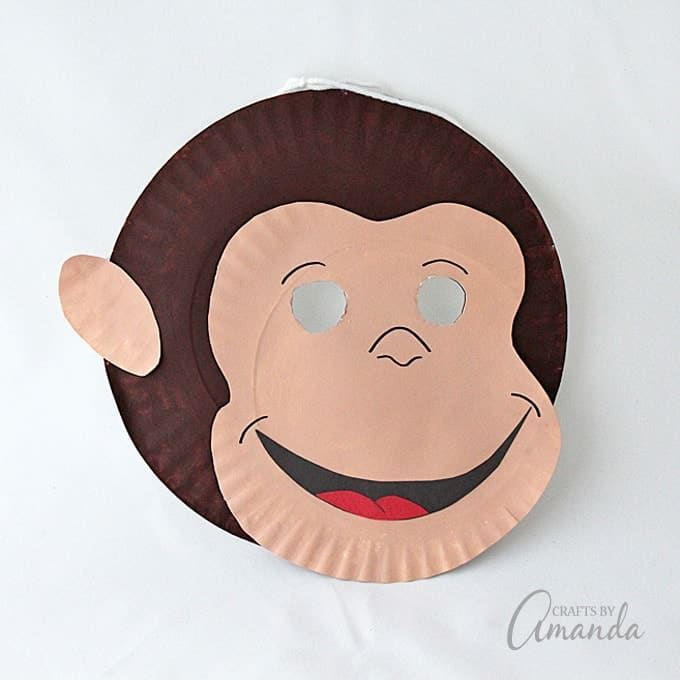The image depicts a detailed kid's craft, resembling the popular character Curious George, against a white background. Centered in the image, there are two paper plates: the back plate painted in dark chocolate brown and the front plate cut and painted to represent the face of the monkey in a light brown, flesh-tone color. The front plate features cutout holes for the eyes, drawn-on nose, and eyebrows, along with a smiling black mouth highlighted by a red tongue. An ear is carefully cut from the same light brown plate and glued onto the dark brown plate, adding to the craft's three-dimensional aspect. Completing the charming monkey's face, small squiggly lines are drawn. The craft appears to function as a puppet or mask, with the eye cutouts allowing it to be held in front of the face. At the bottom of the image, in the lower right-hand corner, the logo "Crafts by Amanda" is visible, indicating the creative source of this engaging project.